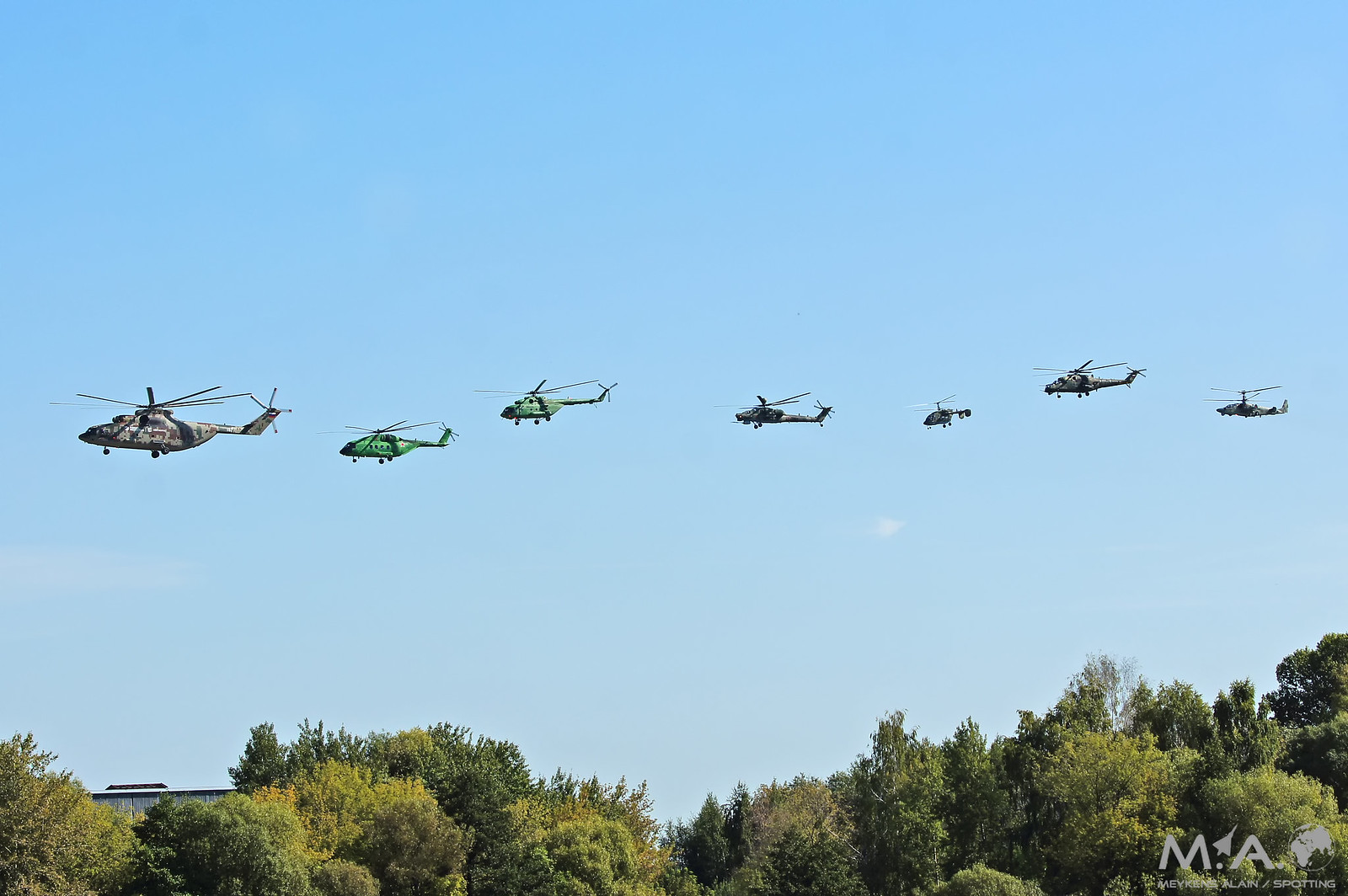The image showcases seven military-style helicopters, predominantly green with some being grayish-black, flying in formation across a clear, bright blue sky with only a few thin clouds. Below the helicopters, a lush forest of deciduous trees expands, the tree line forming a gentle valley midway through and then rising again. On the left, the top of a building peeks out from the trees. In the bottom right corner, there is a gray watermark with the letters "M.A." and between them, a small jet graphic. A white planet Earth is also part of this logo, though interpretations of whether there is also a helicopter or space shuttle included vary.